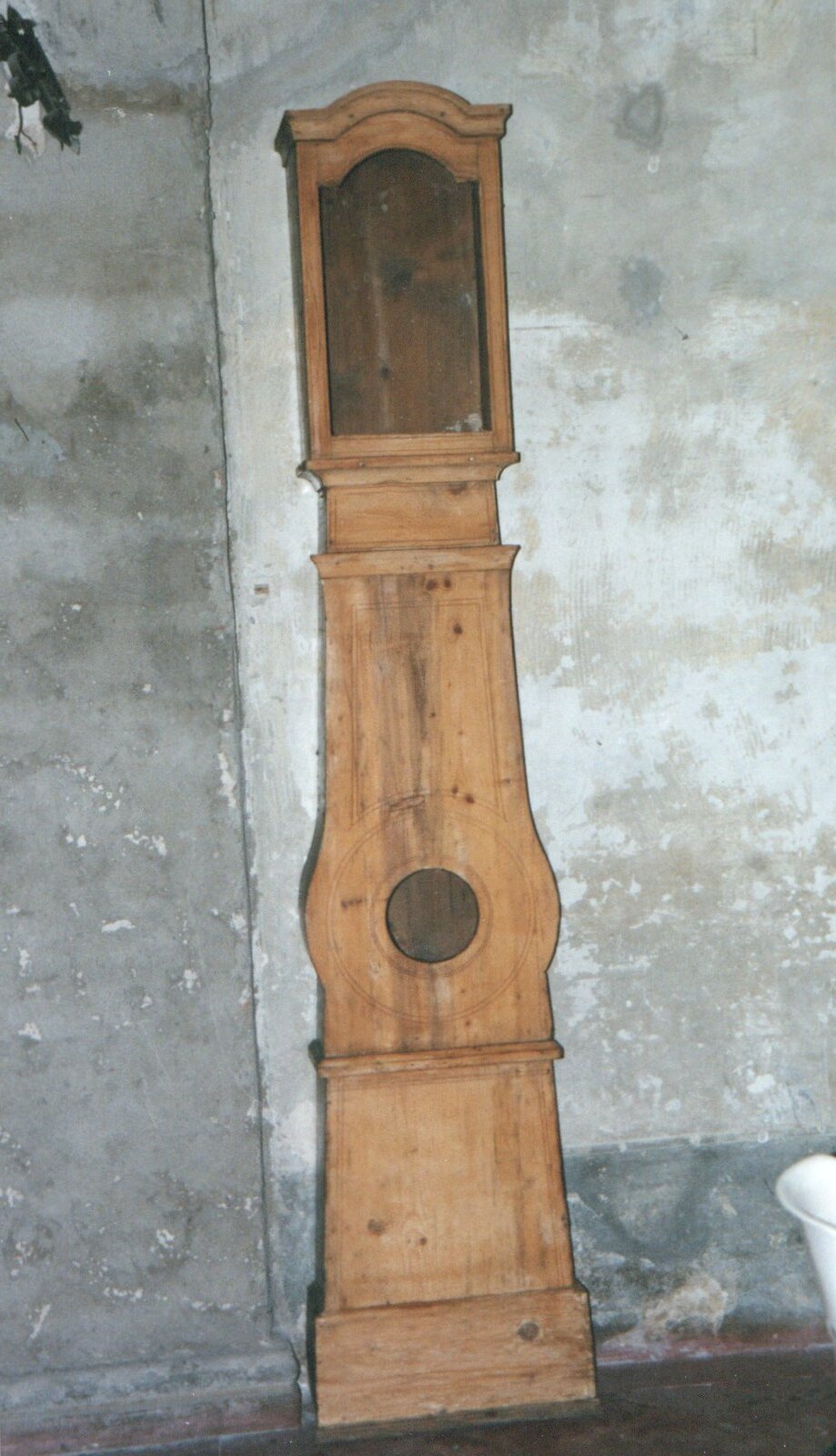The image showcases an old-fashioned stand-up pendulum clock situated in what appears to be an abandoned house. The clock, devoid of a traditional clock face, features a wooden body that forms its structure and supports its upright stance. Through its glass pane, the interior mechanisms are faintly visible, adding to the vintage aesthetic. The surrounding wall, bathed in a grayish-white hue, appears faded and worn, indicative of age and neglect. The wall's texture and color evoke a sense of antiquity, almost resembling a drawing in its dilapidated state. In the background, there is a partial view of what seems to be a small section of a toilet, further emphasizing the air of abandonment and disrepair. The overall scene is steeped in a nostalgic, ghostly charm, capturing the essence of a bygone era.